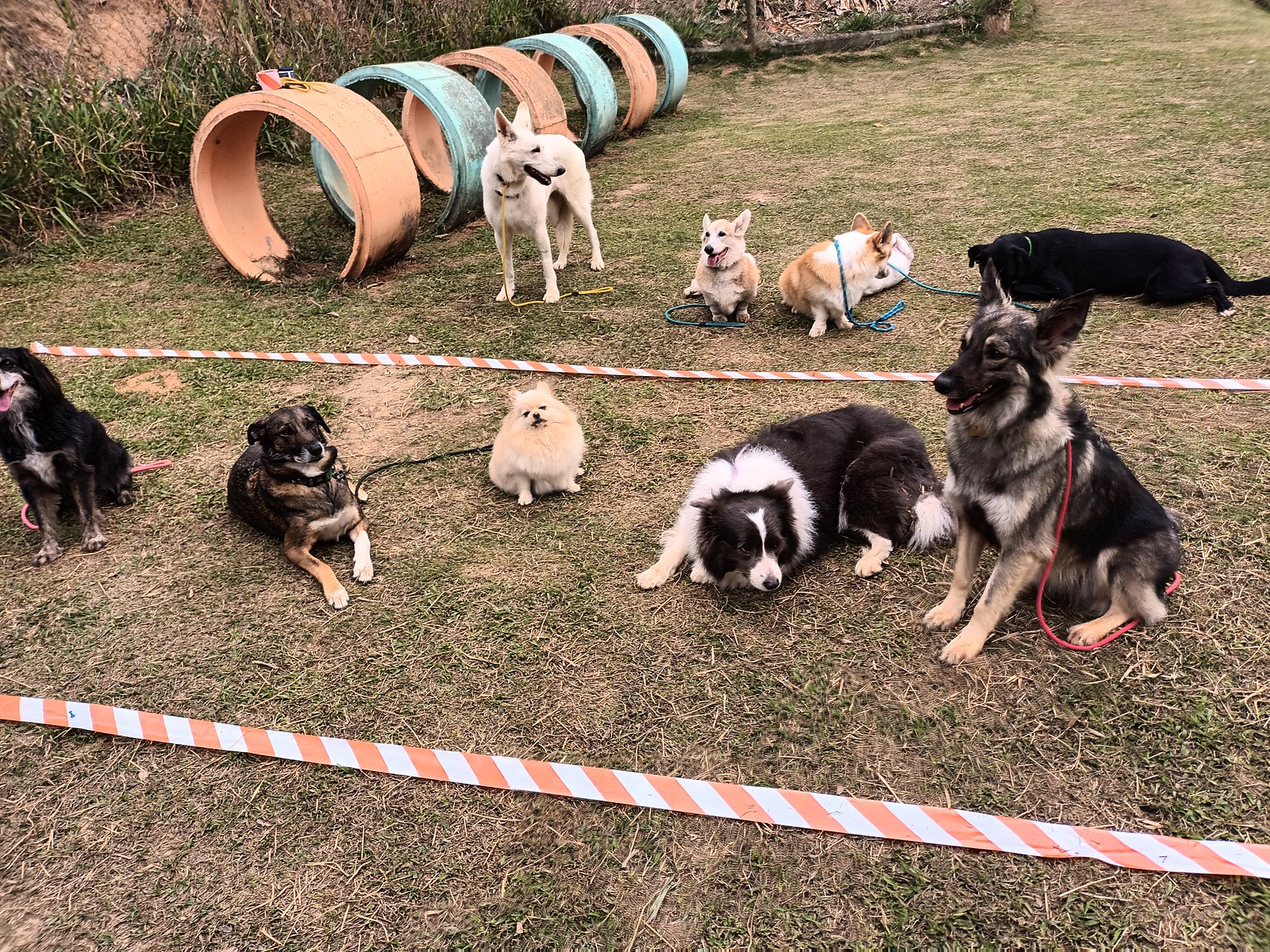This color photograph captures a lively scene of a grassy field, dotted with patches of dirt, and bathed in bright daylight. The main focus is on a variety of dogs, totaling around nine, sprawled calmly across the largely cut-down grass and dirt surface. The image is framed horizontally, allowing a comprehensive view of the scene. 

In the background, to the back left, a chain link fence is visible, partially obscured by overgrown weeds and longer grasses. Adjacent to the fence, there are six agility tunnels or hoops, about two to three feet tall, alternating between vibrant orange and light blue hues. A white and orange checkered tape runs horizontally across the ground.

The foreground and middle ground feature an array of dogs of different breeds, some with leashes trailing beside them. To the left, a Border Collie with a pink leash is partially out of frame, and next to it, an Australian Shepherd Mix lies down, gazing off to the side. A Pomeranian stands alert, facing the camera with a black leash by its feet. Another Border Collie lies with its head on the ground, and beside it, a German Shepherd is looking off to the left with a red leash around its neck. In the background, near the agility tunnels, a Black Lab and two Corgis rest on the grass, while a large white German Shepherd stands nearby. 

The detailed depiction of leashes, the varying colors of the agility tunnels, and the precise positioning of each dog contribute to the vibrant and dynamic nature of this photograph, suggesting a setting such as a dog show or an exercise park.